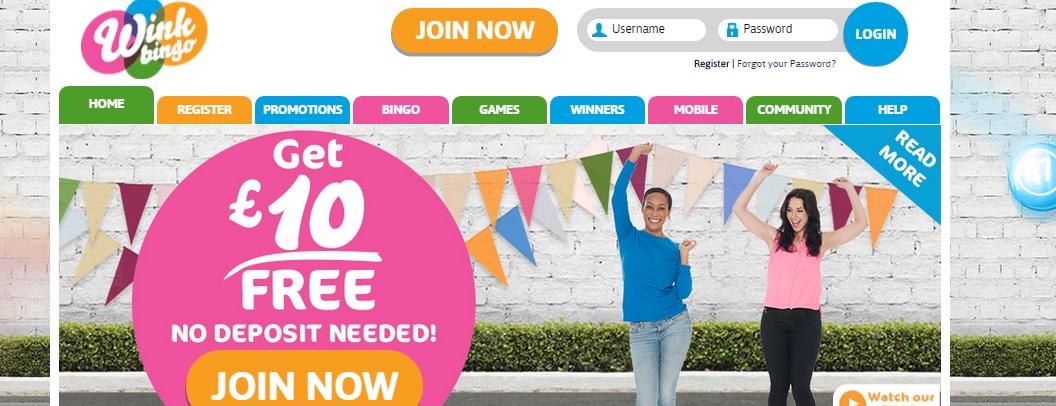A promotional image for an online bingo platform features a vibrant scene with several elements. In the foreground, two women are celebrating; one is wearing a blue shirt and light stonewashed jeans, with her arms raised in excitement. She is Black. The other woman, who is white with long dark hair, is wearing a pink tank top and black shorts, also caught in a moment of joy with her hands up. Above them, colorful flags on a string add a festive atmosphere to the scene. 

To the right of the women, there is a blue ball and the number "1" displayed on the wall. At the bottom right, an orange play button with the text "Watch Now" invites users to engage further. Additionally, a pink circle highlights a special offer reading "Get $10 Free – No Deposit Needed." 

The background hints at further features, including "Join Now," "Username," "Password," "Login," "Register," "Forgot your password," "Promotions," "Bingo Games," "Winners," "Mobile Community," and "Help." The phrase "Read More" is partially visible near the lower part of the image.

Overall, the image is designed to attract attention and encourage users to participate in the bingo platform with a lively and engaging visual appeal.